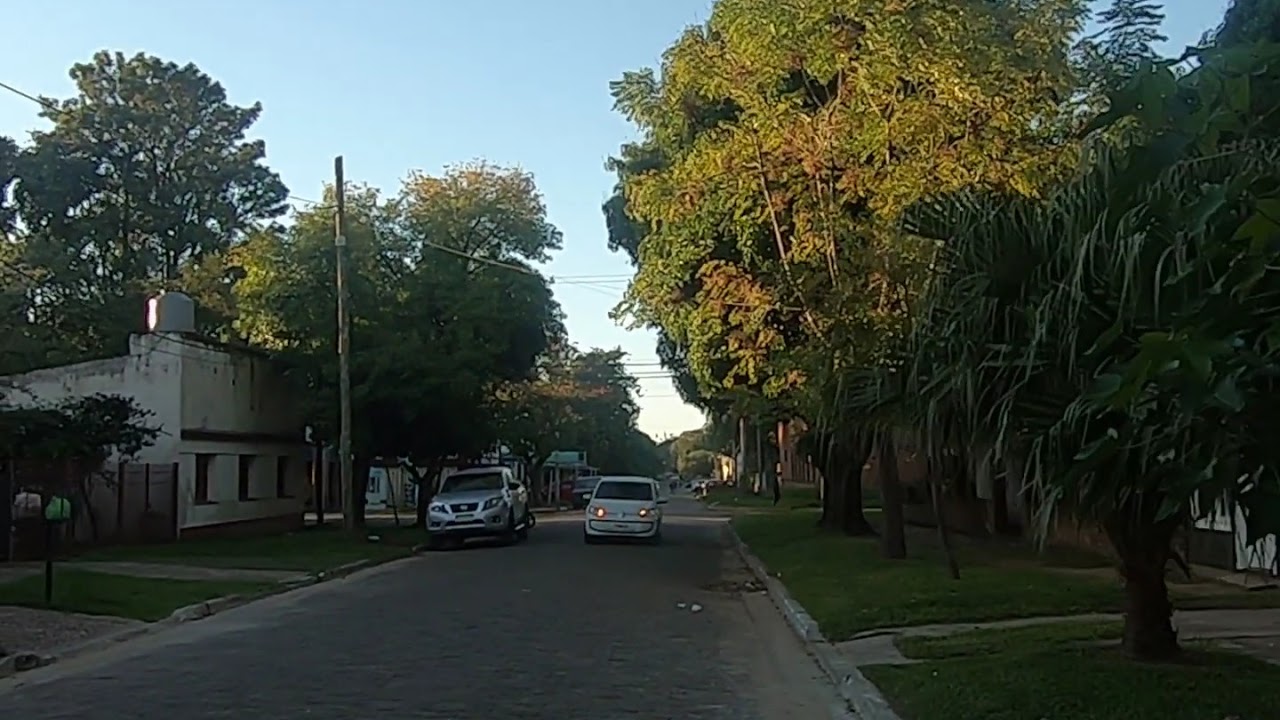This photograph depicts a somewhat rundown residential street at sunset, characterized by a couple of cars and various buildings. Centered in the image is a white van with its headlights on, driving down the middle of a road that shows signs of disrepair. Alongside this van, a gray vehicle, possibly a Jeep or Volvo, is parked on the left side of the road. 

To the left, an old, worn-down white building with black bars on its windows suggests an unclear purpose, possibly industrial or some sort of small storefront. On the right, beyond some large, exotic trees, lie a few houses and apartments hinting at a working-class neighborhood. The buildings and the sidewalk also appear neglected.

The scene is enriched with the presence of utility poles and electrical wires crisscrossing above, capturing the essence of an everyday neighborhood. The top of the trees is faintly illuminated by the setting sun, casting long shadows and signaling the end of the day. This creates a serene, yet slightly melancholic atmosphere, as the photograph vividly contrasts the dilapidated surroundings with the natural beauty of the glowing sunset.